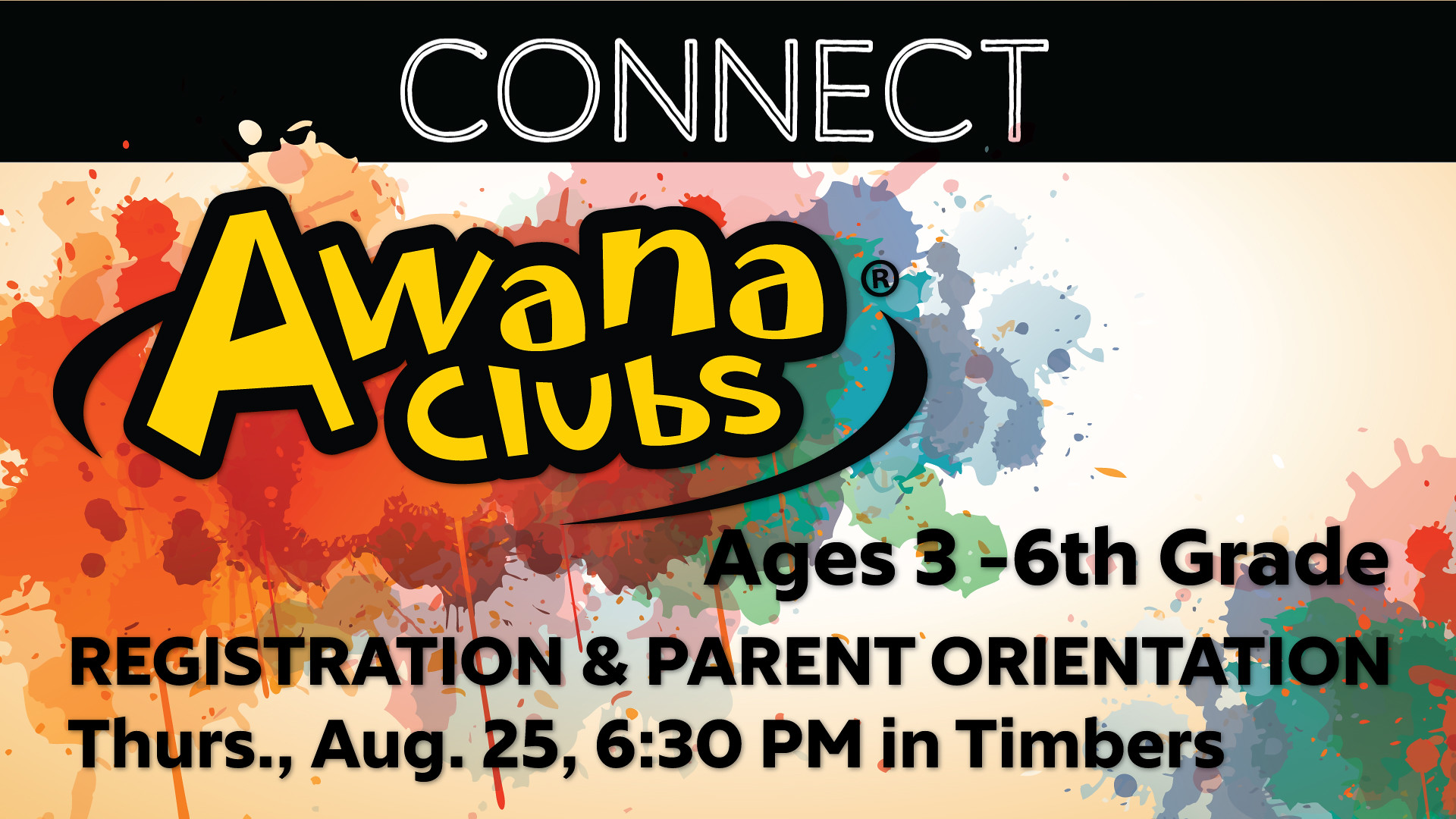The image appears to be an advertisement for a church club, specifically promoting Awana Clubs. The background of the ad is a light peach color, adorned with splashes and splotches of various colors including green, blue, peach, red, and a darker red. At the top of the advertisement, a black bar features the word "CONNECT" in white, stencil-outlined letters, making the text stand out prominently. Below this, the logo for Awana Clubs is displayed in large, bold yellow cartoonish text outlined in black with black interiors in the spaces of the letters, flanked by black swishes reminiscent of a Nike insignia. The lower section of the ad includes black text detailing that the club is for ages 3 through 6th grade, and provides information about registration and a parent orientation. This event is scheduled for Thursday, August 25th at 6:30 p.m., and will take place in Timbers.